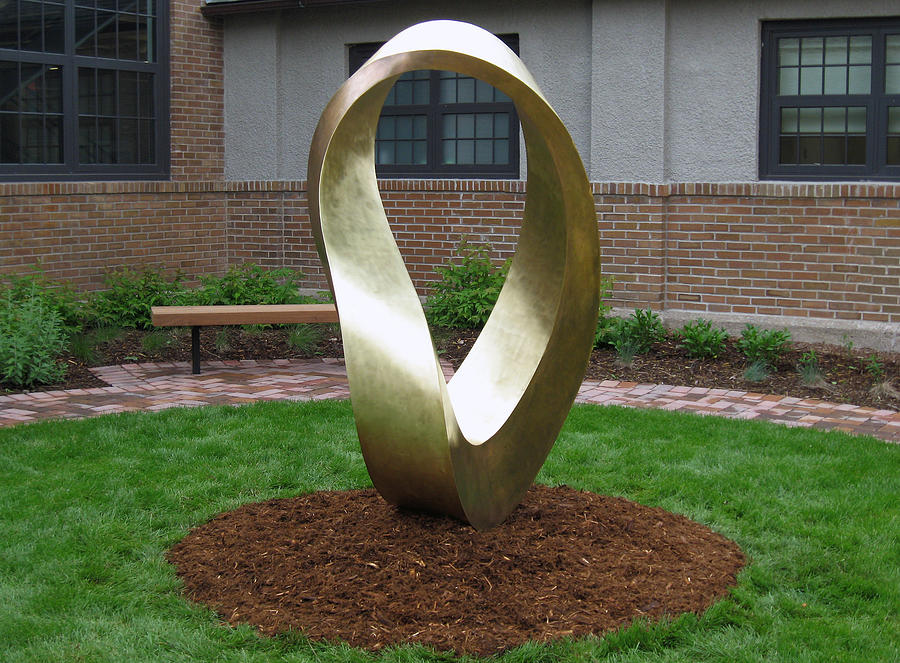The photograph captures a vibrant courtyard set against a building that features a mix of brick and stucco walls, with three large black-framed windows. In the foreground, a meticulously maintained grassy area encircles a central display of brown mulch. At the heart of this setting stands a striking gold-painted statue that conjures images of a Mobius strip. This towering sculpture rises at least six feet and is distinguished by its twisted, tubular structure that loops and bends with an almost impossible elegance. Surrounding the grassy centerpiece is a brick pathway that also features a wooden bench, offering a place to admire the artwork. Encircling the courtyard, a variety of bushes and plants add to the lush greenery, creating a harmonious blend of nature and art.